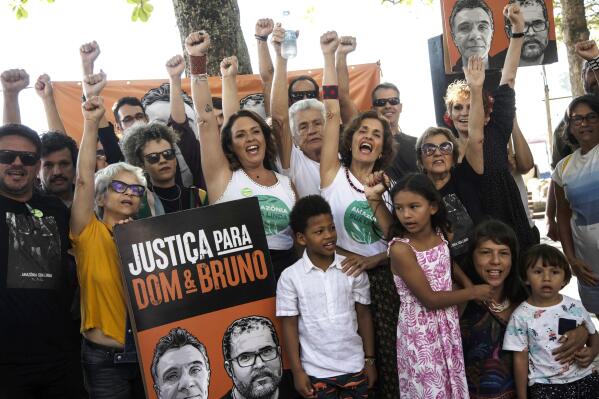This vibrant, full-color photograph captures a powerful moment at a protest held outdoors during the day. Around a dozen people of diverse ages and ethnicities are present, standing beneath the canopy of brown-trunked trees with green leaves. The crowd is united in solidarity, with adults raising their right fists high, and some also raising their left fists. In their hands, they hold posters featuring black-and-white images of two men, Dom and Bruno, alongside the bold text "Justica para Dom e Bruno" printed on a light brown, white, and black background.

The individuals are dressed in a variety of clothing, including black shirts, white tank tops with green centers, and more distinct pieces like a yellow shirt on a woman with black glasses, a pink and white dress on a girl, and a white dress shirt on a boy. Despite the variety in their attire, the message is clear and unified. The scene is framed by trees, capturing the essence of the protest that calls for justice for Dom and Bruno, with the participants looking directly at the camera and emphasizing their cause with their raised fists.